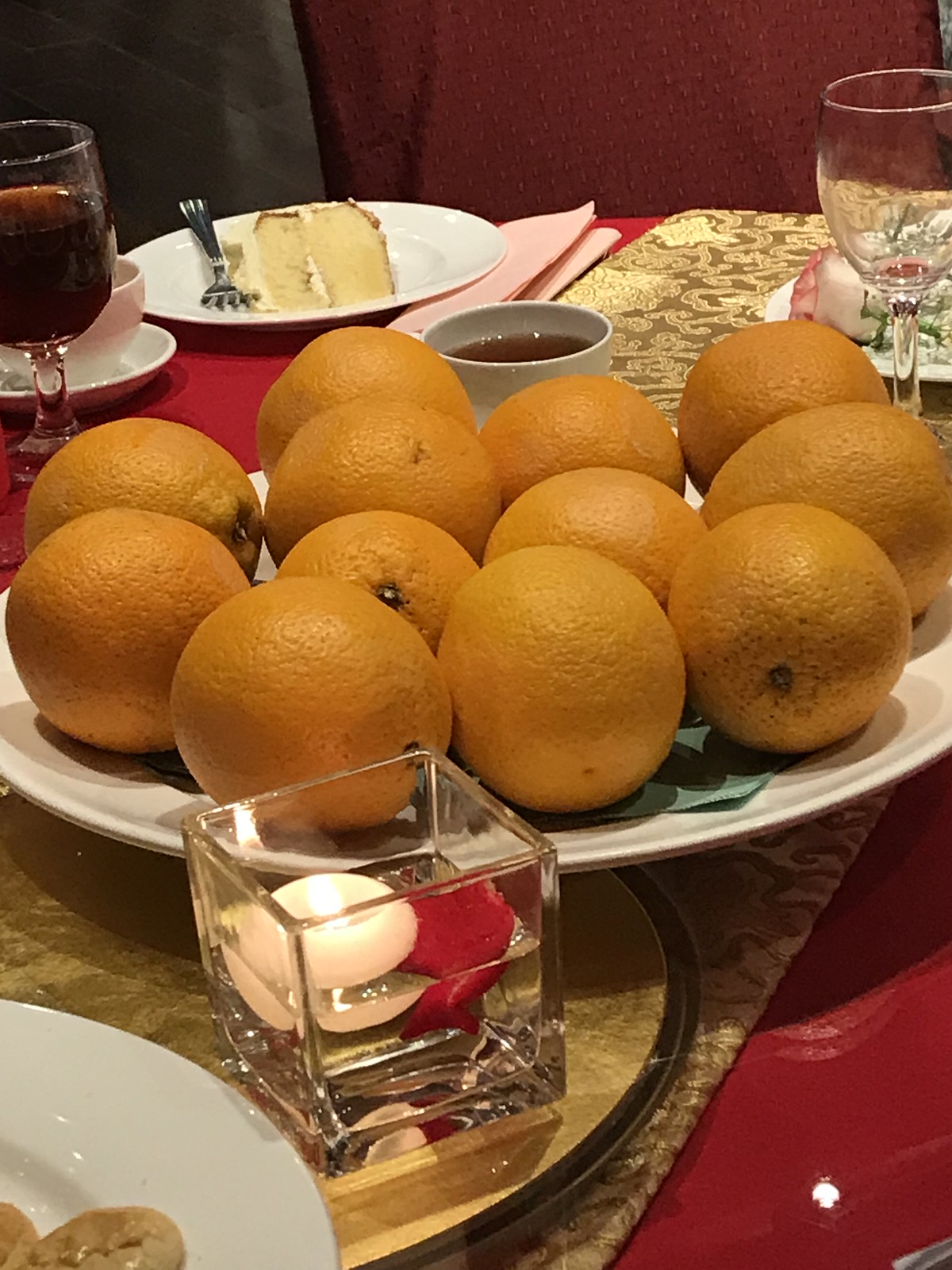In the center of this kitchen table photograph, there is a white plate holding 12 various-sized oranges, which are placed on a mint green napkin. The table features a beige-gold patterned runner with a red edge running across a red tablecloth. In front of the plate of oranges, there is a square glass vase containing a floating candle and possibly a red rose petal, illuminating the white object inside. Towards the lower left corner of the image, we see the edge of another white plate with round, brown cookies on it. Directly behind the plate of oranges, there is a grey dish or small cup filled with a dark brown liquid, which could be coffee. On the upper left side, there's a wine glass with red wine and a matching plate with a slice of gold cake with white frosting and a silver fork. Nearby, another white cup and saucer set sits beside it. The upper right part of the image has an empty wine glass and another napkin. The top background appears red with a different texture, possibly an embossed design, and the upper left corner has a section of black fabric.